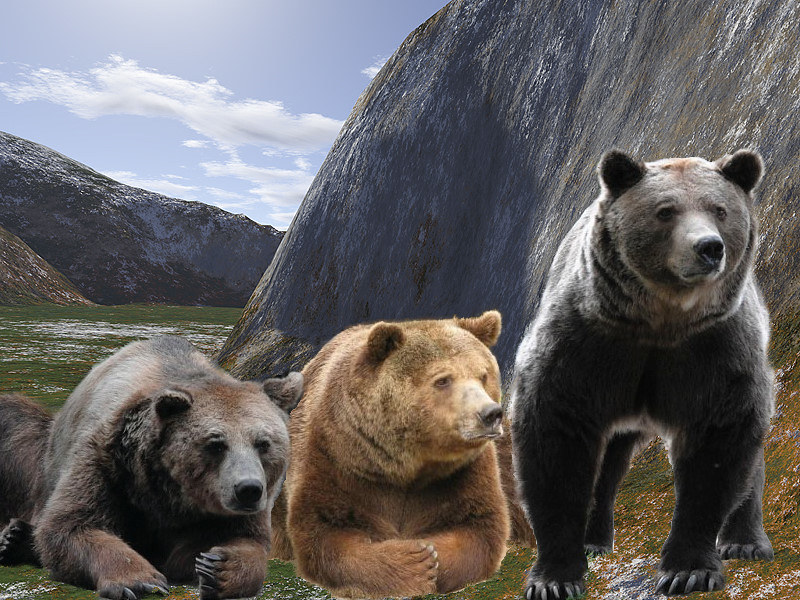The photograph appears to be a photoshopped collage featuring three distinctly different bears set against a meticulously clean and unusual backdrop. In the foreground, on the left, lies a grayish-brown bear with white fur patches, resting low to the ground. The middle bear, with light brown and dark brown fur, is also lying down with its forearms folded over each other. On the right, a black bear with white and gray spots stands on all fours, its sharp claws touching the ground. The bears have been added to a scene that depicts a rocky, mountainous landscape with large rocky formations dominating the background. The ground between the rock formations and the bears is covered in very short green grass, patches of snow, and dirt. The lighting on the bears appears off, lacking shadows, which further suggests that they have been digitally superimposed onto the landscape. The sky features streaky clouds, though much of it is obscured by the imposing rocky hills, which rise up and create a valley-like effect, adding to the scene’s photomanipulated ambiance.